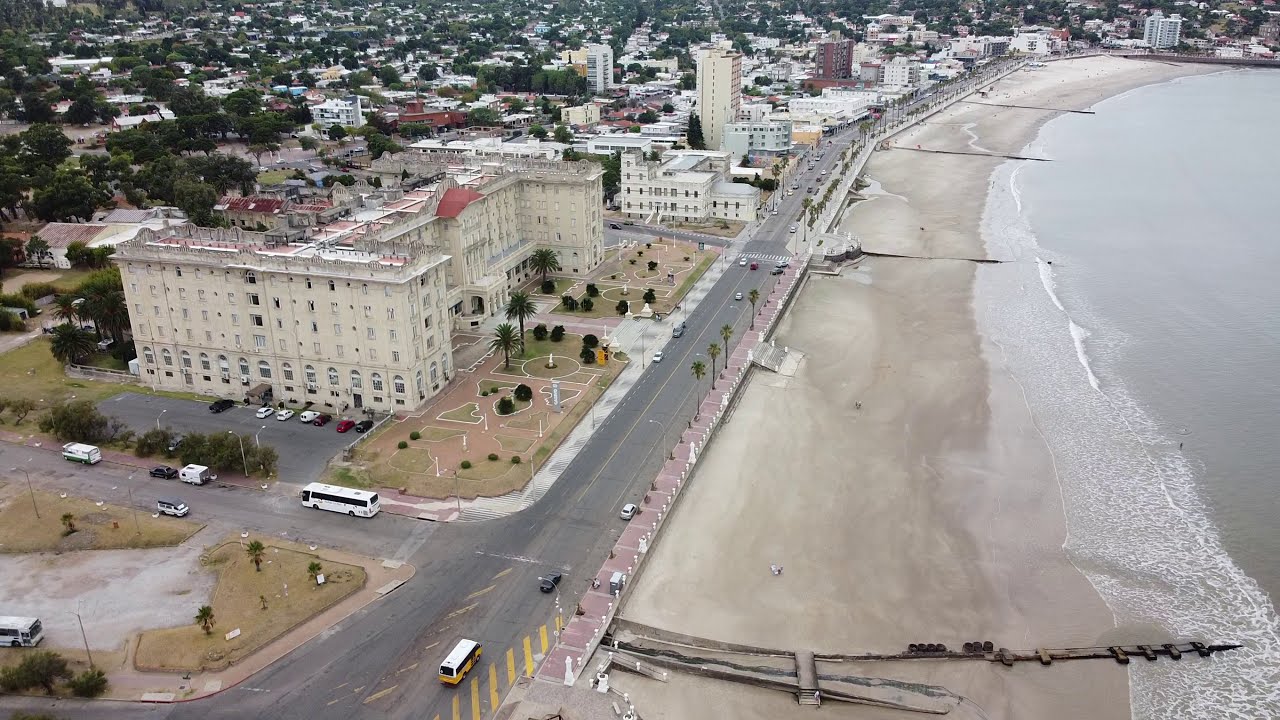This aerial photograph captures a picturesque seaside town stretching across the frame, with numerous notable features. On the right side, the shoreline is dominated by a large beach area with packed, light tan-gray sand leading to gently crashing waves on a pale grayish-blue body of water, giving an impression of a cooler day. The beach extends into piers protruding from a blacktop road running parallel to the coastline. Towards the middle of the image, a sparsely populated sidewalk bisects the beach and a section of the town, where couple of palm trees and a two- to three-lane roadway are visible. 

To the left, the town is densely populated with a variety of buildings partially obscured by patches of green trees. Notably, there is a series of modest-height structures, including six-story white stone condominiums and a large, creamy white building with a significant number of rooms and windows, possibly resembling a hotel. This building features courtyard areas with grass, palm trees, and bushes, and a number of vehicles, including a white bus, are parked around it. A perpendicular road intersects this area, weaving through the verdant patches of land and additional buildings. The upper portion of the image reveals the town’s sprawling extent, filled with numerous green trees blending with the multitude of buildings as far as the eye can see.